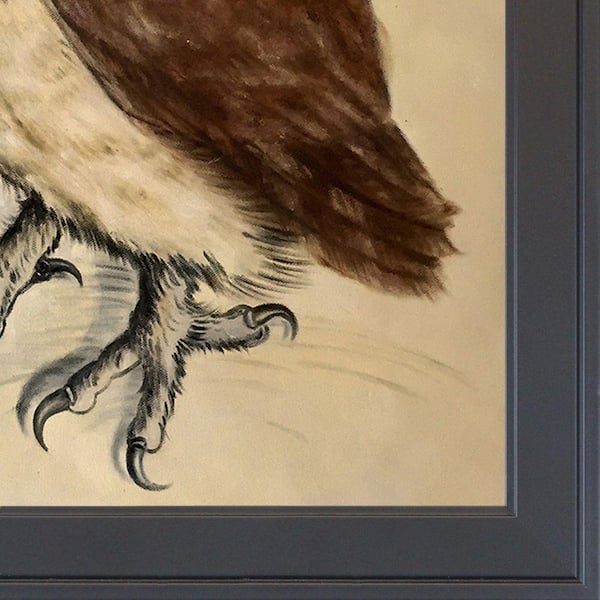This image captures the lower right corner of a framed picture, prominently featuring the talons of a bird, possibly an owl or an eagle. The bird's sharp claws, drawn in black and gray, are visible on three digits of one foot, with a partial view of the other leg. The bird's body has distinct areas of brown and white or beige feathers, depicted in intricate, sharp sketch-like lines. The background inside the frame is a tan color, providing contrast to the bird's dark brown feathers. Surrounding the image is a charcoal gray or black frame, with the mat behind the picture also being tan. The photo is very zoomed-in, emphasizing the detailed textures and colors of the bird and its surroundings.